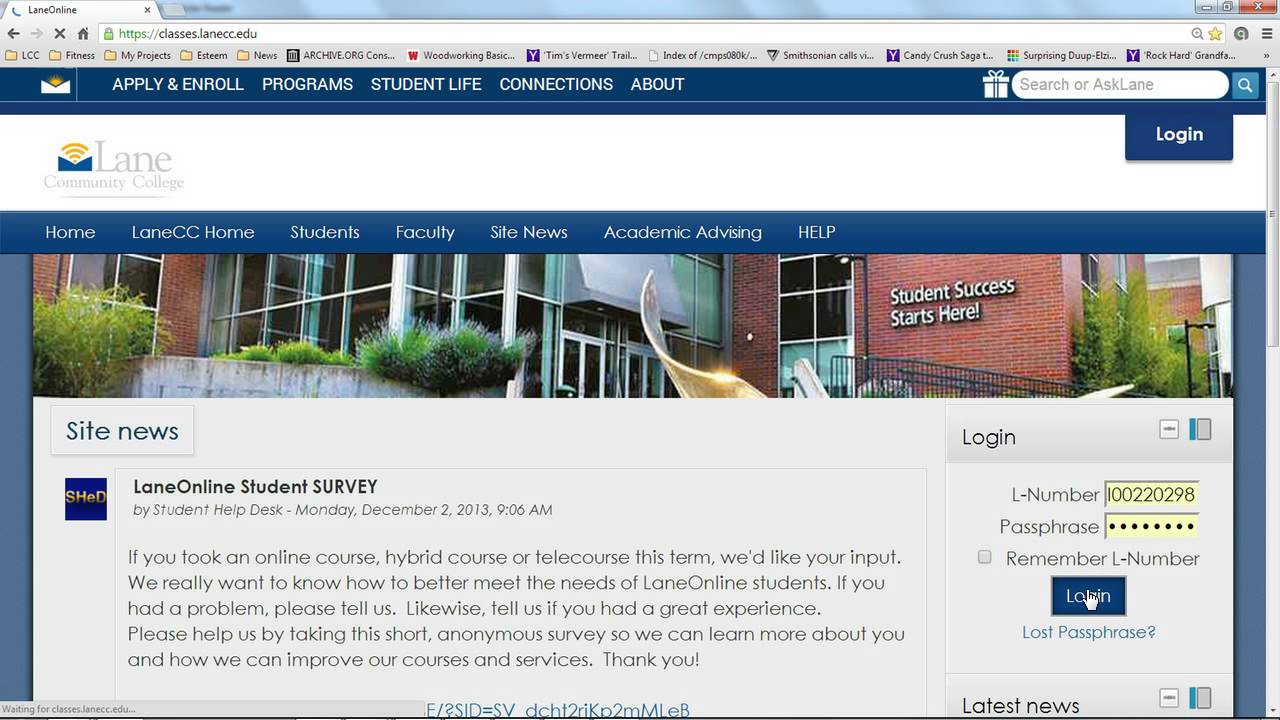This screenshot captures the home page of Lane Community College's website. At the top, you see the browser's address bar and bookmarks toolbar. The page features a blue header bar that includes website navigation sections on the left and a search bar on the right, with a login button situated below the search bar.

Central to the page is Lane Community College's logo, prominently displayed within a white banner. Below the banner, a key photograph showcases a college building with the inspiring text "Student Success Starts Here" emblazoned across it.

The main navigation categories are listed as follows: Home, Lane CC Home, Students, Faculty, Site News, Academic Advising, and Help. Below the main photograph and aligned to the right, there's a login section where users can enter their L number and passphrase to access their accounts. The login button is highlighted by a hand cursor hovering over it.

To the left of the login section, there's a gray box labeled 'Site News', highlighting the latest update: "Lane Online Student Survey", accompanied by some explanatory text. The page also features a gray scroll bar on the right, indicating additional information is available below the visible portion of the page.